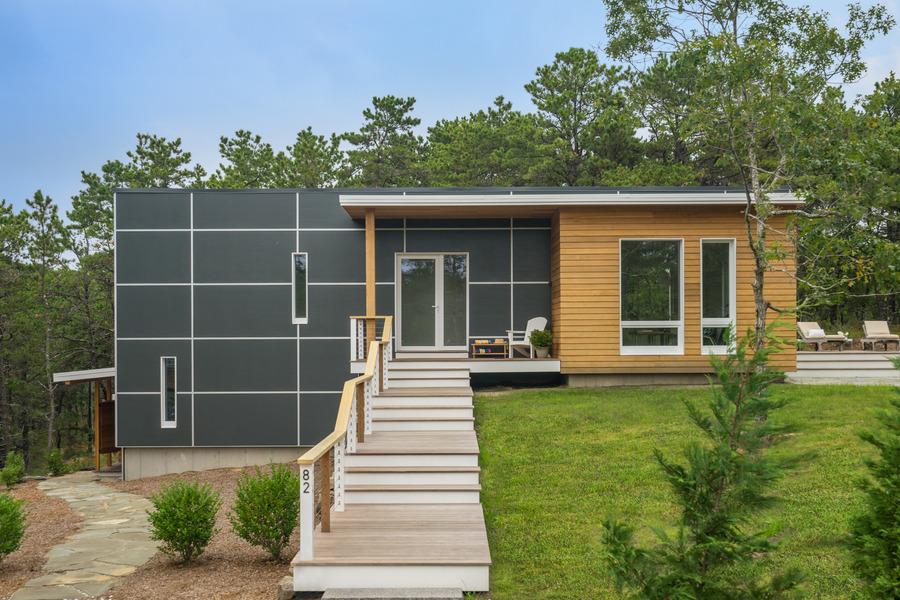The photograph features a striking, geometrically designed modern home characterized by straight, clean lines. The facade prominently displays a dark grey rectangular grid pattern overlaid with a white grid design. To the right of this grid section, a wooden-paneled facade protrudes, adding warmth to the modern aesthetic. The entrance is approached by a shallow wooden staircase consisting of about nine steps, leading up to a glass door sheltered by a flat rectangular awning supported by a rectangular pillar. 

Flanking the house are skinny, vertical rectangular windows that enhance the structure’s sleek look while allowing natural light to filter in. The number 82 is clearly visible as the address on this stylish home. To the right, there is an outdoor patio furnished with two chairs, suggesting a comfortable space for relaxation. The house also boasts a wooden walkway that leads to the front entrance, and a stone walkway curves around to the back of the house.

The setting appears to be tranquil, surrounded by lush green grass, bushes, and well-maintained trees in the background, indicating a rural or forested location. The meticulous landscape complements the modern architecture, creating a harmonious and inviting environment.